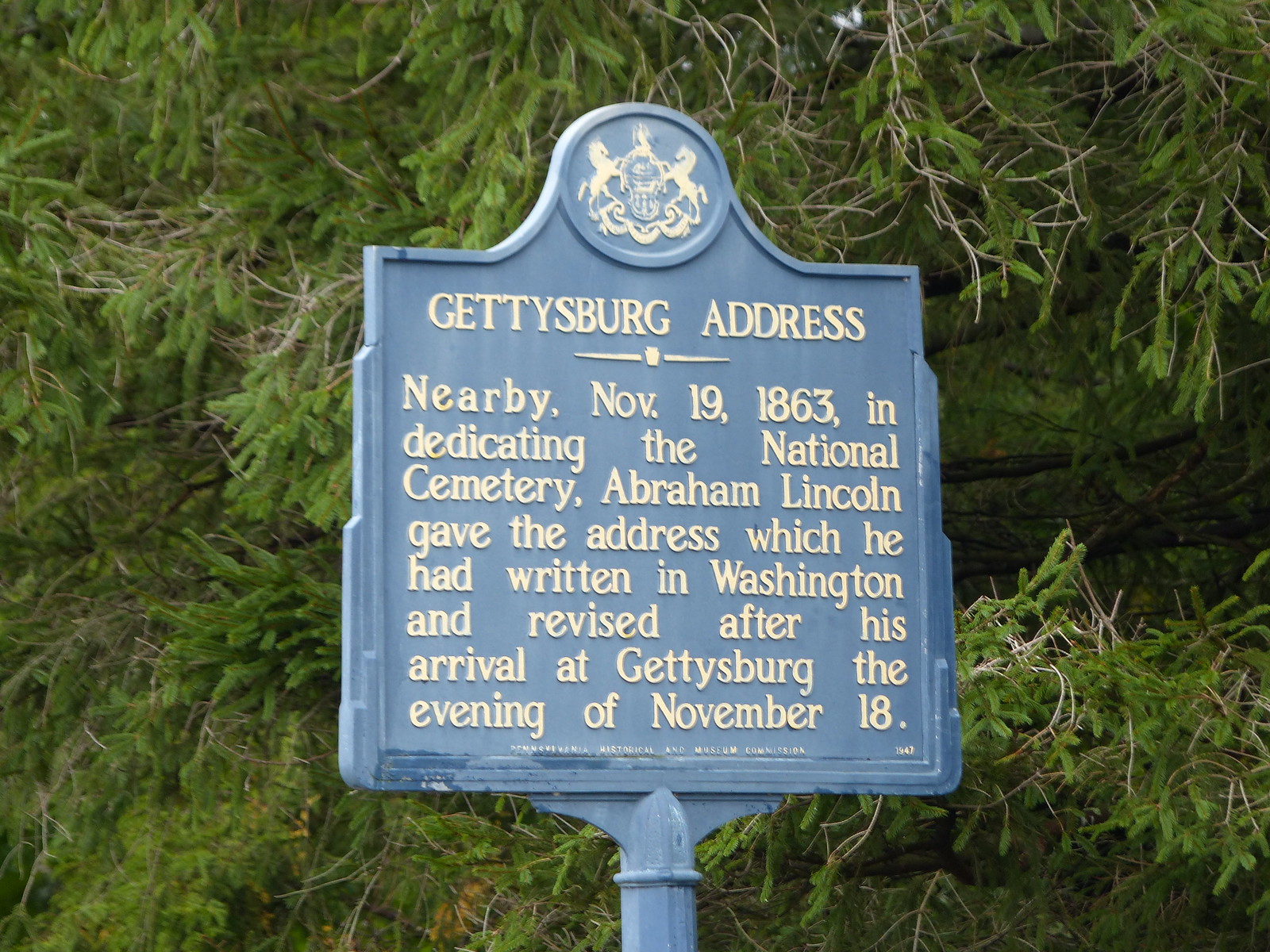This photo captures a historical marker set in a forested area, prominently featuring pine trees that dominate the background. The marker is a blue sign with yellow and white writing, centered on a pole. An insignia at the top depicts two horses touching a globe. The text below the insignia reads: "Gettysburg Address. Nearby, November 19th, 1863, in dedicating the National Cemetery, Abraham Lincoln gave the address which he had written in Washington and revised after his arrival at Gettysburg the evening of November 18th." The surroundings and the focus on the marker suggest this is where the historical event took place.